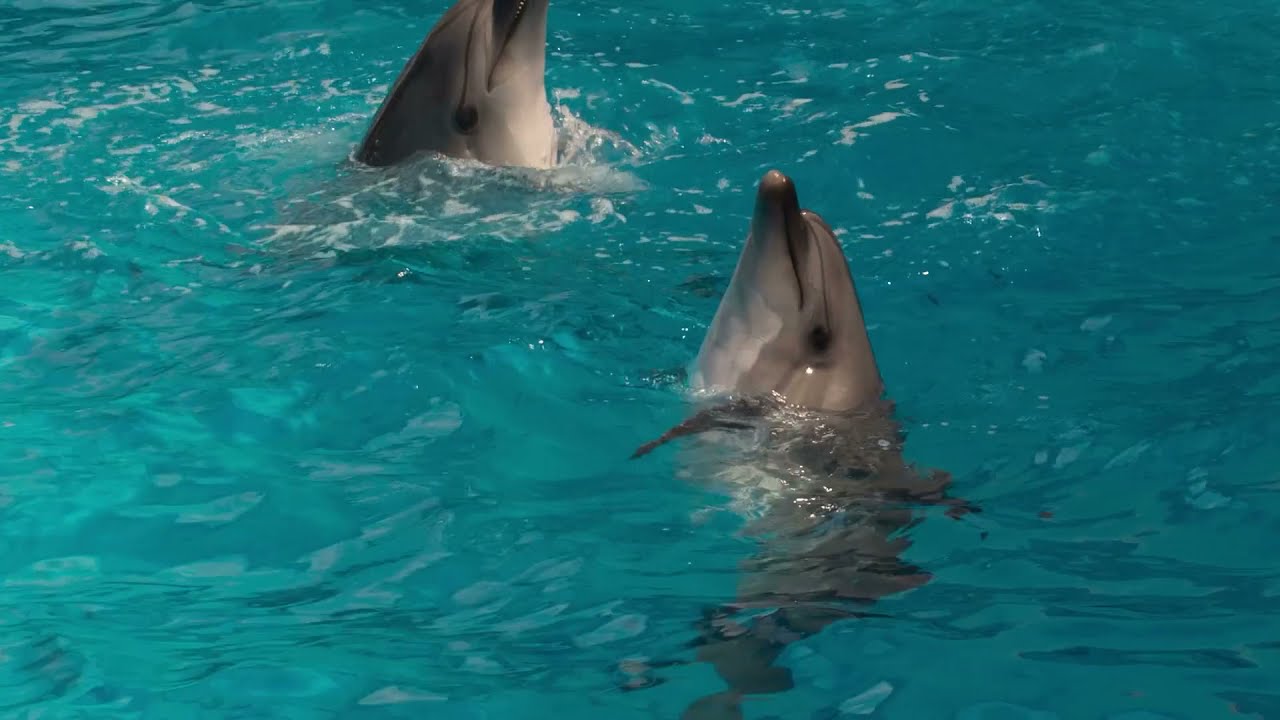In this vibrant and joyful image, we see two playful bottlenose dolphins in a shimmering turquoise-blue pool, likely within a commercial setting such as a marine park or zoo. The water is so clear and clean that their gray bodies, with white undersides and black eyes, appear almost to vanish into it, creating a blurred effect that leaves their heads much clearer than their bodies and tails. The dolphin closest to the middle of the image seems to be preparing to jump, with its head and part of its body above the water. Its mouth is slightly open, while water splashes around both dolphins, creating white foamy areas. This splashing adds a dynamic frothiness to the scene, enhancing their playful and joyous demeanor. The background is entirely filled with the bright turquoise water, emphasizing the controlled and likely artificial environment of their aquatic habitat.